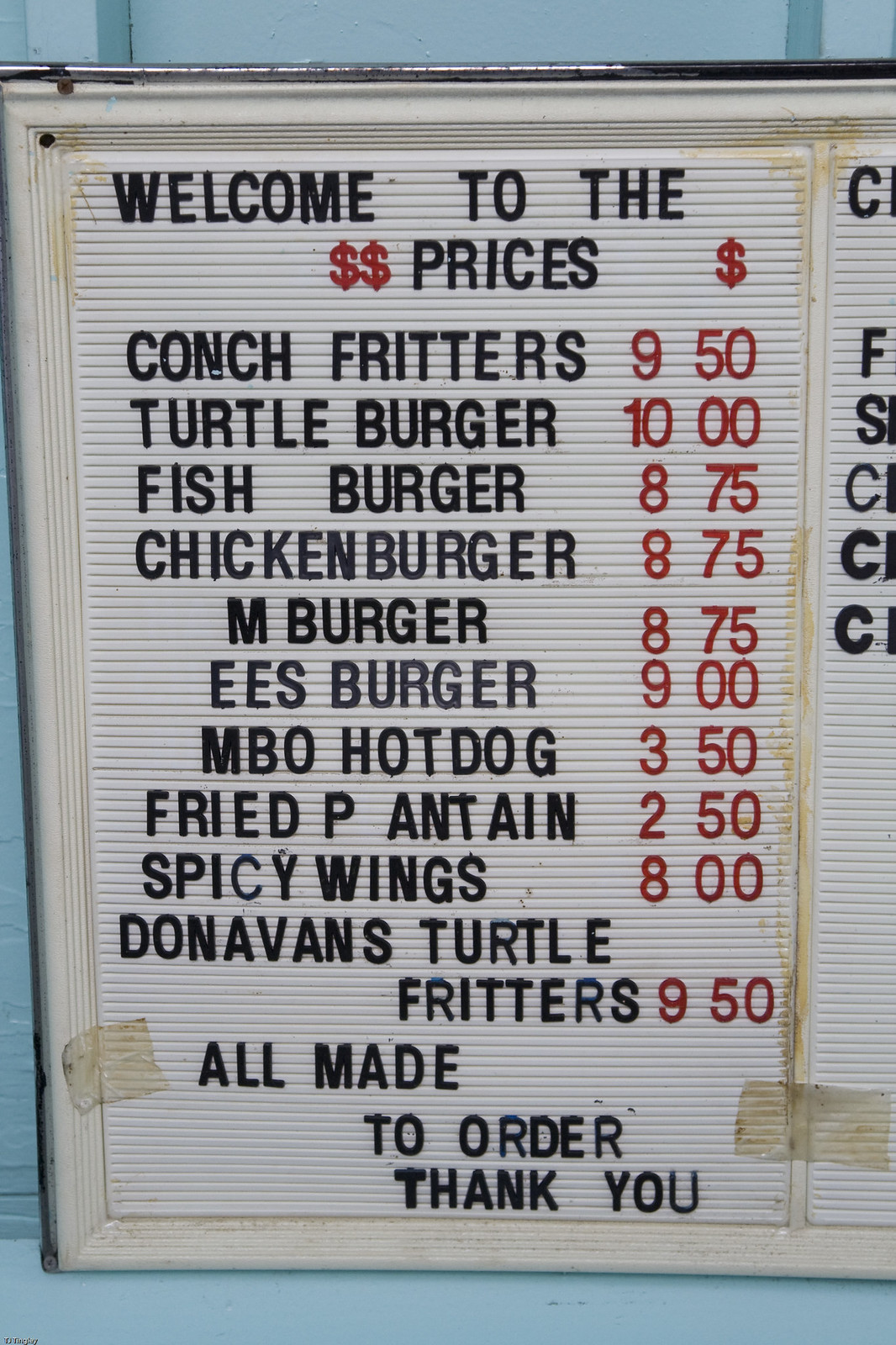In this image, we see a detailed price board, possibly from a carnival or an outdoor event. The sign welcomes visitors with the text "Welcome to the Prices" emblazoned at the top. It meticulously lists a variety of menu items, including Conch Fritters, Turtle Burger, Fish Burger, Chicken Burger, M Burger, E's Burger, MBO Hot Dog, Fried Plantain—although the "L's" in "Plantain" are missing—Spicy Wings, and Donovan's Turtle Fritters. Each item is made to order, ensuring freshness, as noted at the bottom of the list, followed by a courteous "Thank you."

The price board is double-sided, but only the contents of the primary side are visible. The partially obscured reverse shows just the initial letters of unknown items. Each menu item has a corresponding price listed next to it. 

The sign itself is propped up on a ledge that has a distinctive stripe of blue along its bottom edge. To keep the sign secure, pieces of tape are affixed on both sides, with additional strips running down near the middle bottom and along the side edge of the sign. This practical setup ensures the board remains stable and visible to patrons.